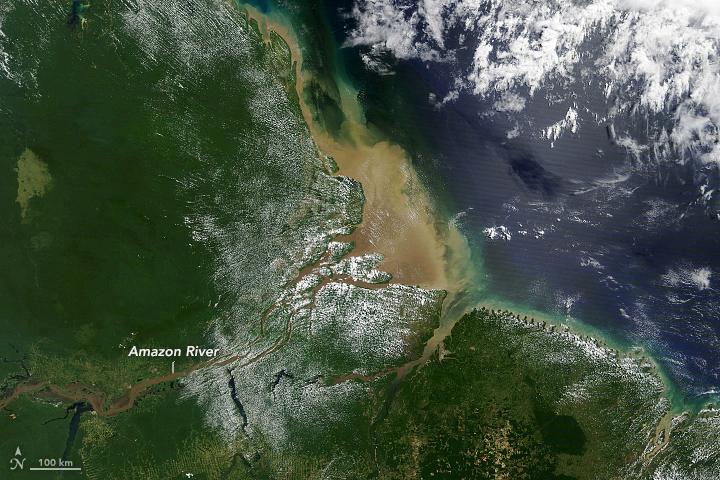This satellite photograph captures a detailed view of the Amazon River as it snakes through the lush, green Amazon rainforest and eventually meets the Atlantic Ocean. The image prominently features the Amazon River as a brown line winding its way across the land. The river is labeled "Amazon River" with a small dash pointing to the brown water. Towards the bottom left of the photograph, a triangle with the letter "N" denotes the direction of north, alongside a scale bar indicating 100 kilometers.

The river's journey is vividly depicted as it twists and turns before dispersing into numerous branches upon reaching the coastline, where it deposits sandy brown sediment into the ocean. This sediment-laden water contrasts with the dark blue of the open sea, which is partly obscured by white cloud cover in the top right corner of the image. As the river's muddy discharge diffuses into the ocean, the water transitions from brown to varying shades of green before blending into the deep blue of the ocean further out. The diagrammatic elements combine to provide a comprehensive understanding of the geography and scale of this incredible natural feature.